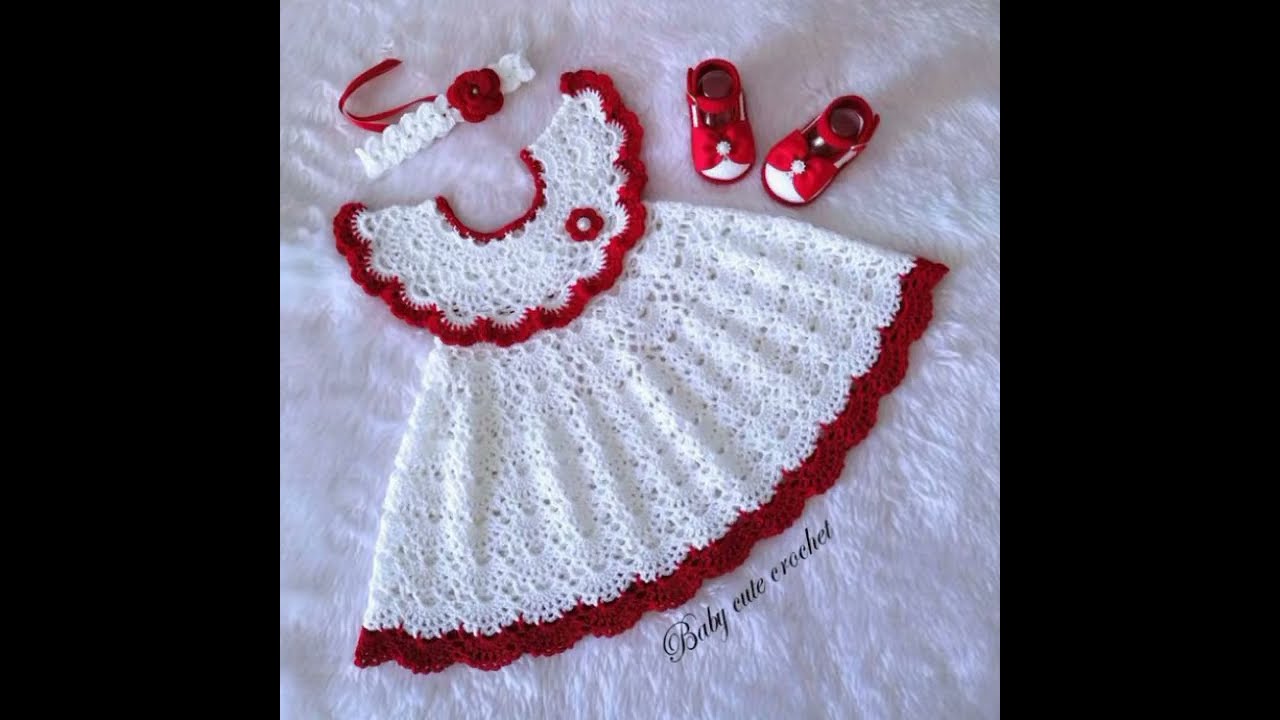The image is a highly pixelated and distorted digital photo with a black and white background resembling a digital mesh or code. In the foreground, there appears to be a yellowish-white short-sleeve shirt and a pair of shorts, possibly laying flat as if on a display or bed. The shorts seem to have frilly bottoms, which might appear sequined or knitted due to the effect on the photo. The image also features red curved lines or marks across it, which resemble spray paint. Overall, the image is blurry, unfinished, and difficult to interpret clearly due to its heavy pixelation.